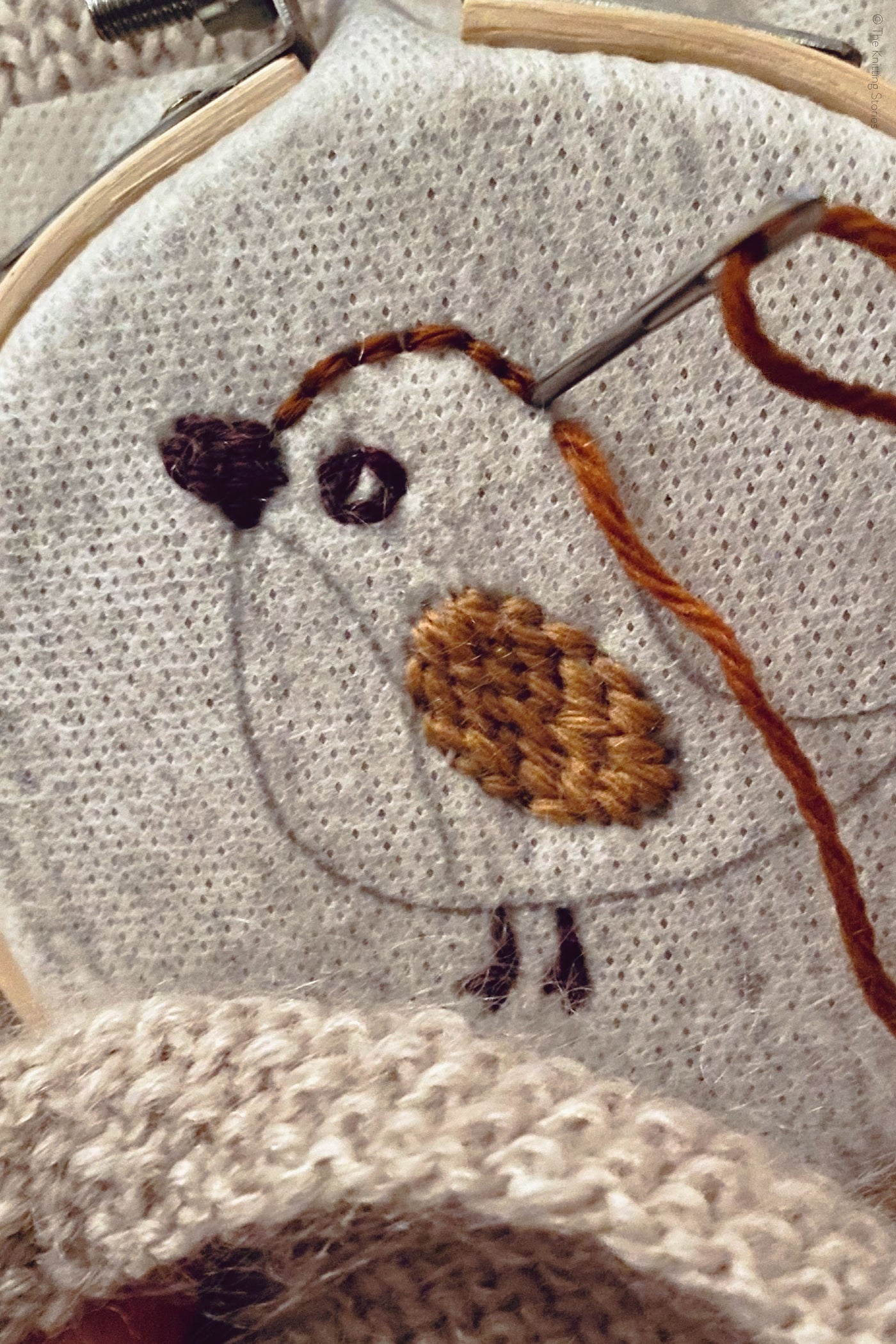In the image, we see an embroidery project in progress within a wooden hoop. The hoop holds a piece of white and gray fabric taunt, dotted with small black holes. A silver crochet needle, threaded with brown yarn, is inserted in the fabric at the center, winding upwards to the right. The emerging pattern depicts a bird, with the head beginning to take shape at the needle's entry point. The bird features a detailed black eye with a white spot, and a rounded black beak facing right. Its wings are embroidered in brown, while the legs, stitched in light brown, extend from the body. A heavier thread arches below the bird, adding texture to the design, and beneath this, there's a section of brown fabric visible. The bird’s chest is outlined separately, indicating a different color to be added later. The precise stitching captures the intricacies of the bird, promising a beautifully detailed finish.